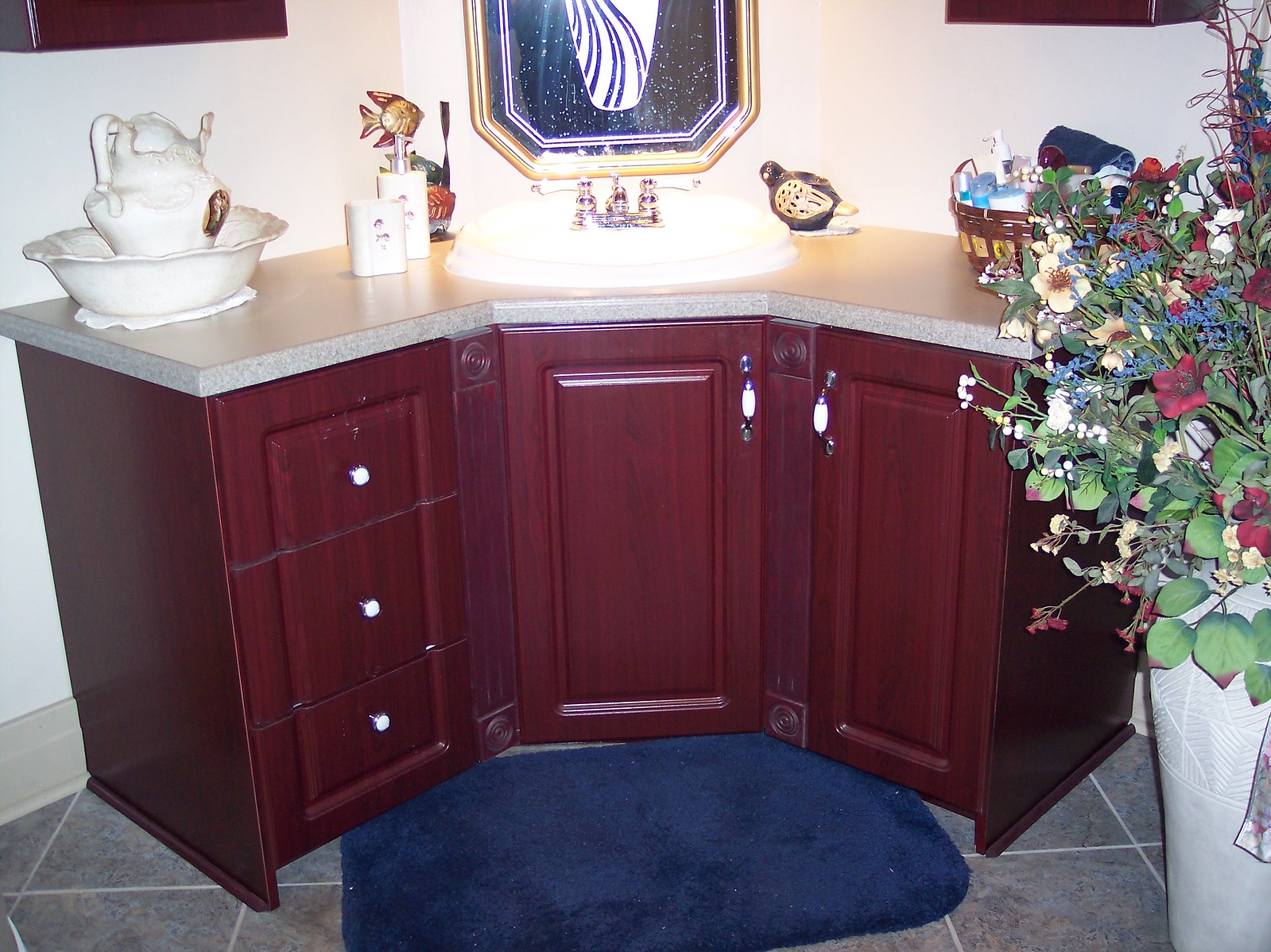The image depicts a retro-themed bathroom styled with elements reminiscent of 1980s and 90s design aesthetics. The focal point is a corner sink crafted from rich mahogany wood. The sink features golden faucet handles, adding a touch of opulence. Above the sink is a somewhat dirty mirror encased in an ornate gold frame. The bathroom's left corner houses a petite white water fountain adorned with a sculpted swan that appears to be spitting water. To the right of the sink, there's a basket brimming with various lotions and hand creams. Further to the right, a bouquet of artificial flowers stands; despite being fake, they appear to be wilting, lending an intriguing contrast to the scene.